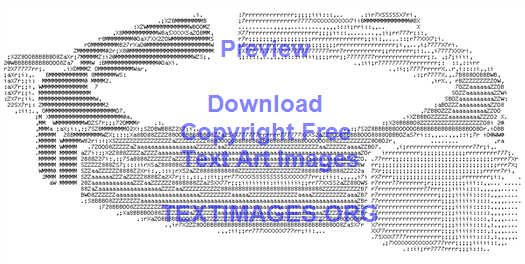The image, created using typewriter or computer-generated symbols, depicts a three-dimensional ring structure resembling the Ubuntu logo. This intricate design combines various characters and text to form a detailed black and white graphic. The ring features three cross-sectioned parts, each with a smaller ring encircling the center, showcasing varying shades from dark on the left to light on the far right. Positioned beneath the ring and towards the right is a smaller cylinder. Overlaid on the graphic is blue text stating, "Preview, Download copyright-free text art images, textimages.org," indicating the source where similar text art can be obtained. The entire composition is displayed on a white background, emphasizing the precision and artistry of the text-based design.